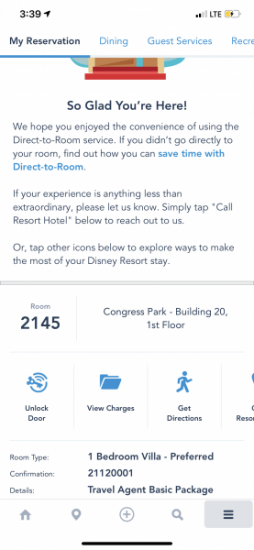The image displays a vertical mobile screenshot of a reservation page with a white background. It is divided into three main sections: the top navigation bar, an upper text portion, and a bottom text and icon portion.

In the top left corner, the time is displayed as 3:39, alongside a battery icon indicating it's about half full. Connectivity symbols for LTE and Wi-Fi are also visible. The top banner includes four tabs: "My Reservation," "Dining," "Guest Services," and a partially visible word, "RECRE," cut off at the right. The "My Reservation" tab is selected, indicated by bold text.

Below the top section, the page warmly welcomes the user with the message, "So Glad You're Here," followed by three paragraphs and a prominent blue link reading, "Save Time with Direct to Room." 

The bottom portion is delineated by a thin gray line. It provides the room information: "Room 2145 at Congress Park, Building 20, first floor." Beneath this, there are four interactive icons labeled "Unlock Door," "View Charges," "Get Directions," and a fourth icon that is partially cut off on the right.

Further details follow, including the room type, confirmation number, and additional specifics, although these are not fully visible in the screenshot. At the very bottom, there are five icons aligned in a row, separated by a thin black line.